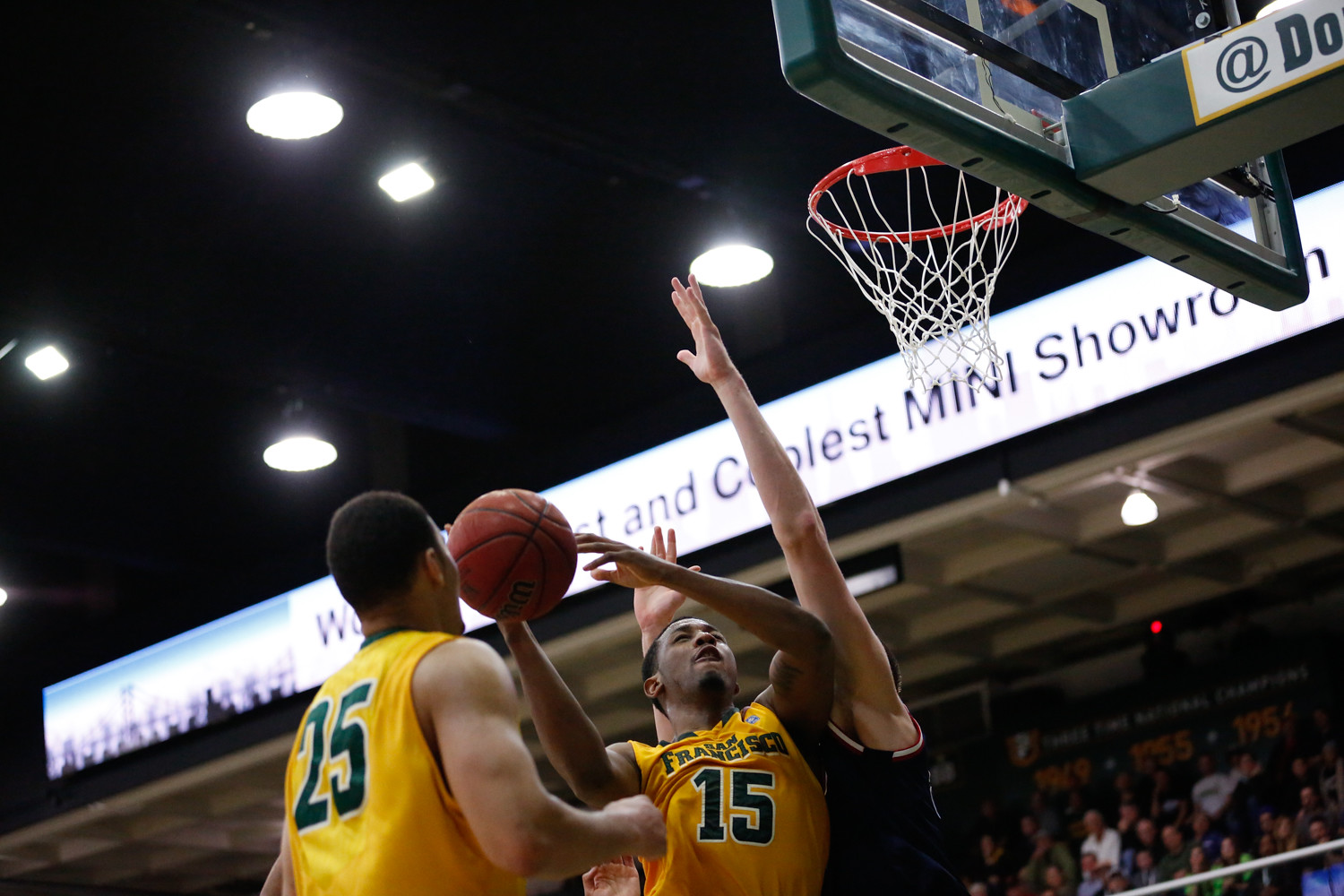This photograph captures a dynamic moment in a basketball game, featuring three players near the basket. The central focus is a player clad in a yellow jersey, numbered 15 on the front, emblazoned with "San Francisco," as he prepares to shoot the basketball. A teammate, in the same yellow jersey with the number 25 on the back, is positioned to the left, identifiable by his short black hair. Both players are opposed by a defender in a solid black jersey, whose raised arms obstruct the shooter, with the basketball poised between his hands and the hoop. The hoop, with its transparent backboard, is situated in the upper right corner of the image. Behind the players, a white banner reads, "Coolest Mini Showroom," though it is partially obscured. Spectators fill the background, seated and attentively watching the game, under the illumination of multiple white lights affixed to the black ceiling above.